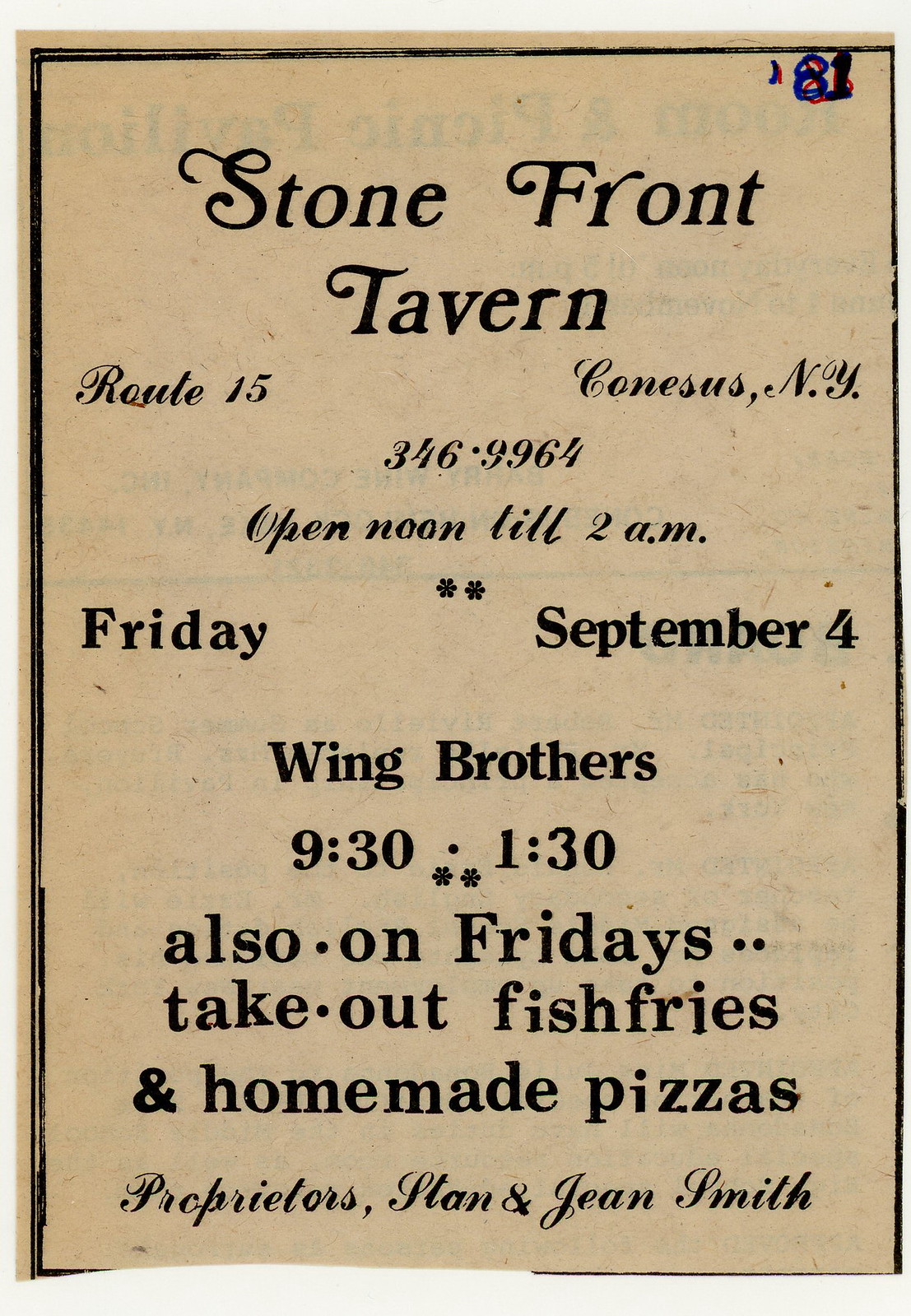This image features a rectangular advertisement or flyer with a cream-colored background and black text. At the top right corner, the number "81" is displayed in blue, black, and red colors. The flyer includes a black line border. The text on the flyer reads: "Stonefront Tavern, Route 15, Conessus, NY. Phone number: 346-9964. Open from noon till 2 a.m. 

On Friday, September 4, enjoy live music by the Wing Brothers from 9:30 p.m. to 1:30 a.m. Additionally, on Fridays, we offer takeout fish fries and homemade pizzas. Proprietors: Glenn and Jean Smith." The flyer has a handwritten aesthetic.